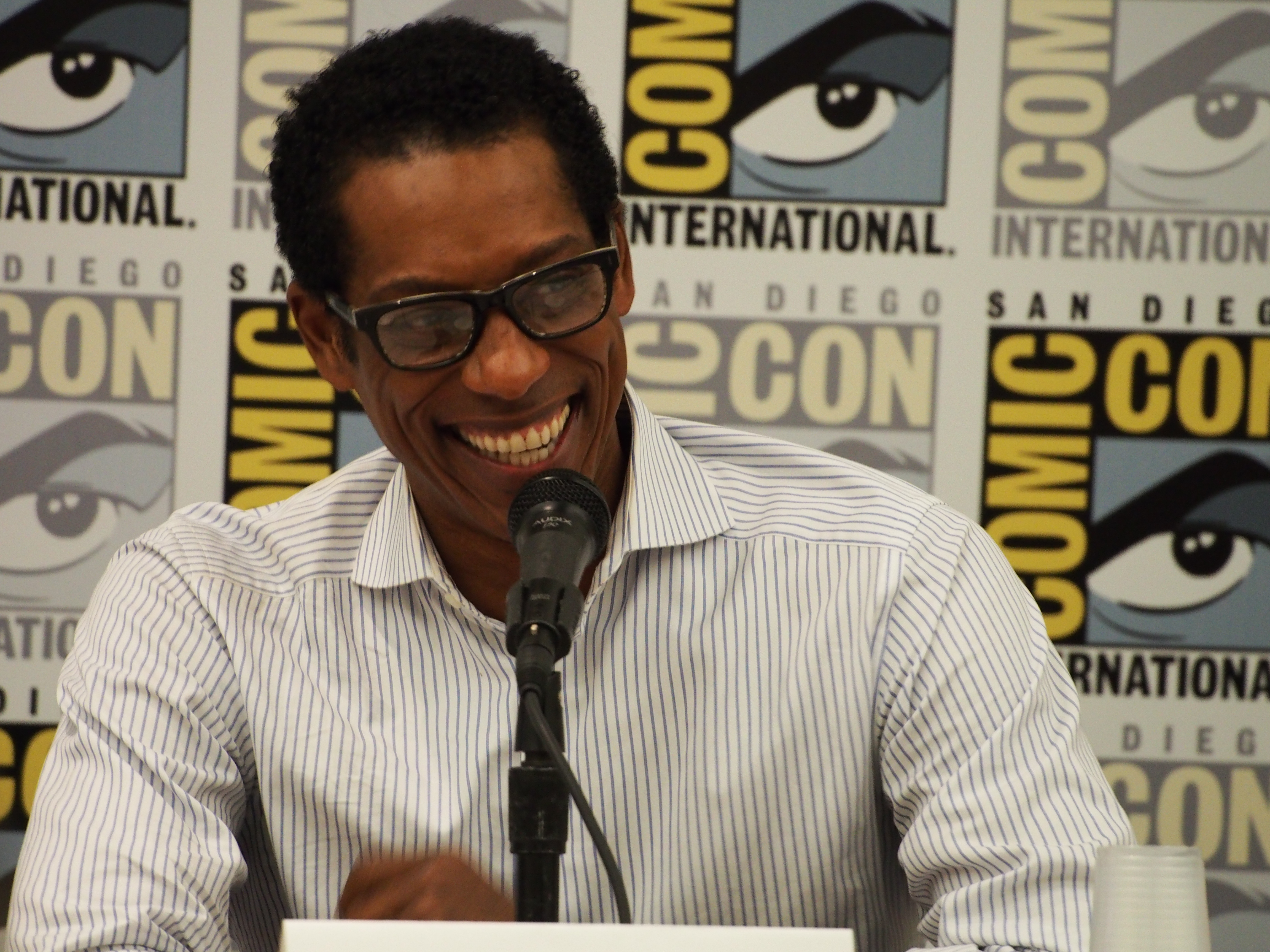This image, captured at Comic-Con San Diego International, features the renowned musician Herbie Hancock. He is seated on stage, smiling broadly and laughing, clearly enjoying the moment. He sports black-rimmed prescription glasses and a white long-sleeved shirt adorned with blue pinstripes. A black microphone is positioned right in front of his mouth, suggesting he is part of a panel discussion. Behind him, the Comic-Con logo and banner are prominently displayed, repeating over and over. In front of him, a name tag and what appears to be an upside-down plastic cup are visible on the table. Hancock's left hand is raised, possibly in mid-gesture, adding to the animated and joyful atmosphere of the image.